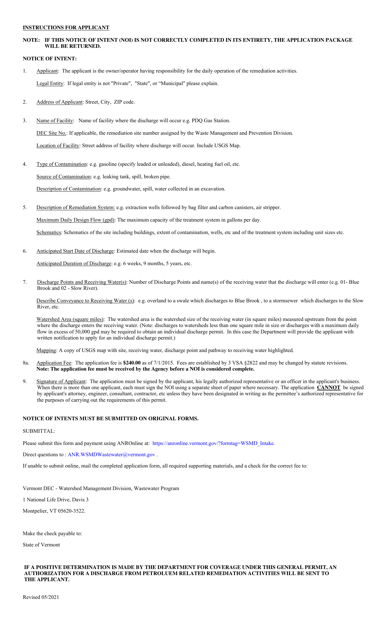The image in question is extremely small, making it difficult to discern any specific details or text clearly. The only identifiable elements are a white background with some black text, which appears to include sections labeled "Instructions for Applicant" and "Notice of Events." Unfortunately, the text is too minute to be readable, rendering the content effectively unintelligible. This has been part of an ongoing issue with images presented recently, but this particular instance is notably the most challenging due to the complete lack of legibility. There are no additional events or updates, such as a soccer game, to provide further context or content. Hopefully, future images will be more legible and easier to analyze.